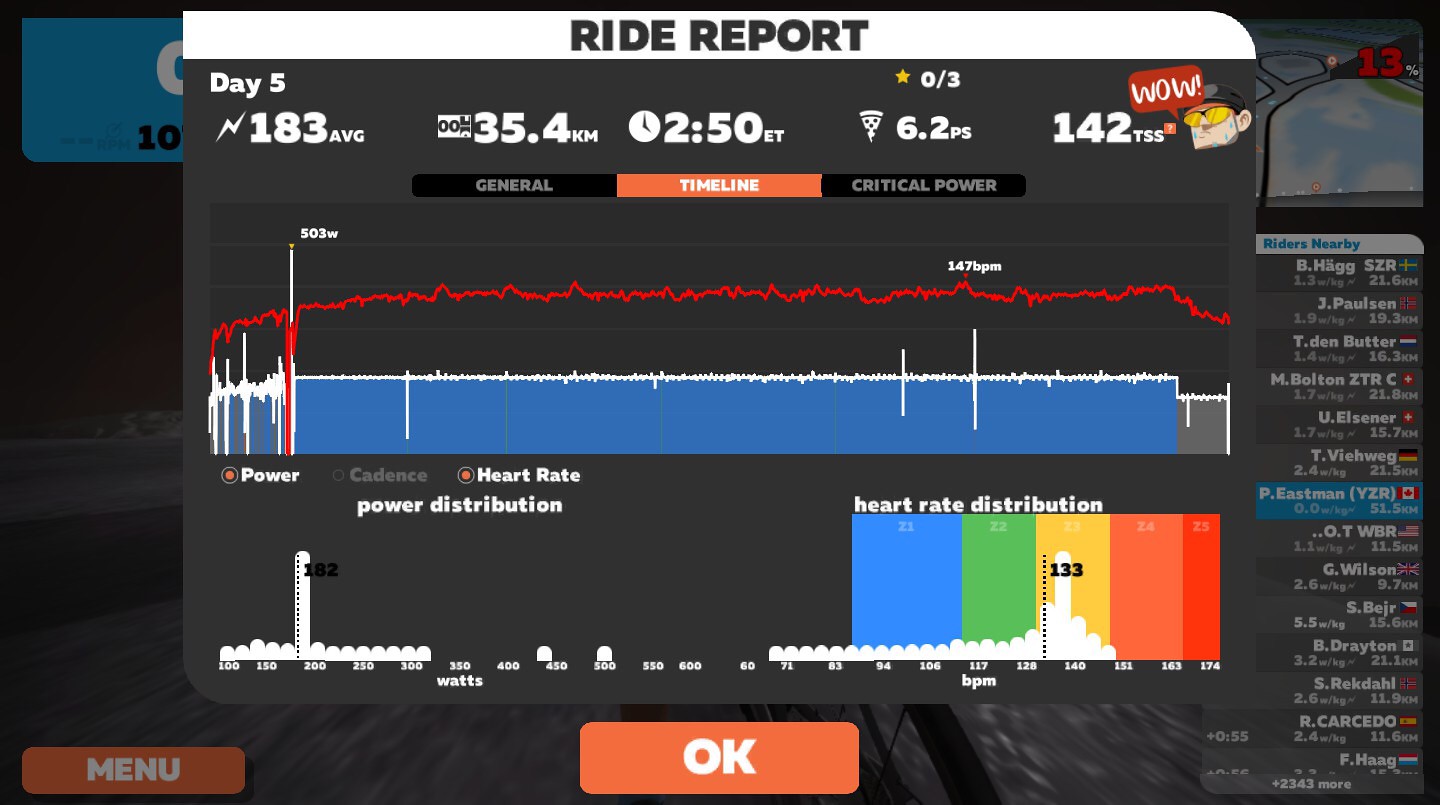The image appears to be a detailed screenshot from a health and fitness application that tracks cycling performance. Central to the interface is a comprehensive Ride Report set against a gray background. The report is prominently labeled "Ride Report" in black text on a white bar at the top. Below, the black area features key ride statistics: "Day 5, 183 average BPM, 35.4 kilometers, 2:50 ET, 6.2 PS, and 142 TSS," accompanied by a lightning symbol and a character with a speech bubble saying "Wow."

The interface includes multiple graphical representations of the data. A blue chart with white and red lines appears in the middle, displaying a detailed heart rate and power distribution over time. Beneath this, there are two additional bar charts: one labeled "Power Distribution" with white bars, and the other "Heart Rate Distribution," featuring colored bars in blue, green, yellow, orange, and red. 

On the right side of the image, a partially grayed-out screen shows a list of nearby riders, each identified by their initial, last name, and national flag. An orange button marked "Menu" is located on the left side of this section. Anchoring the bottom of the image is another prominent orange button with white text that reads "OK."